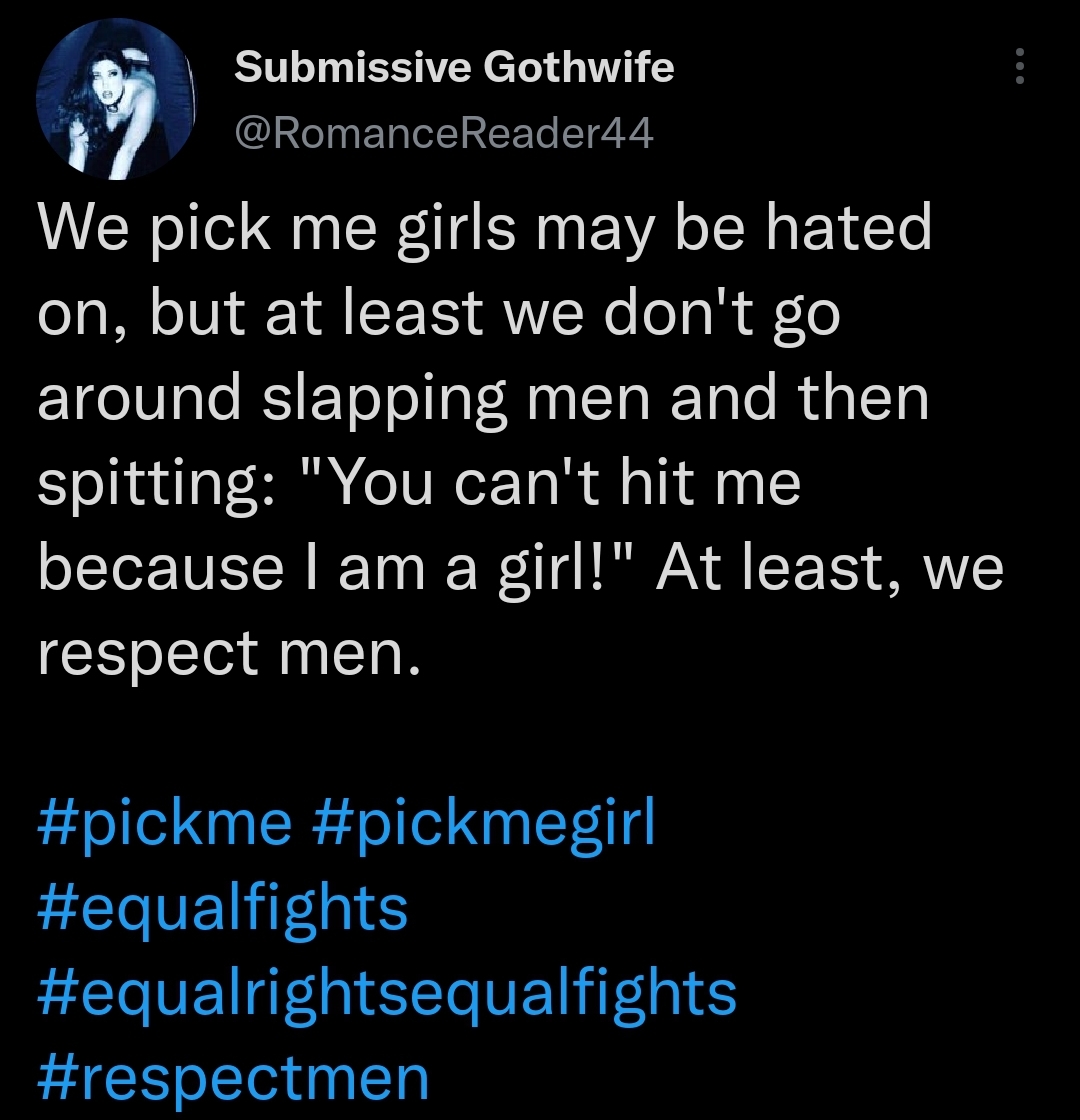The image is a screenshot of a social media post, presumably a tweet, by a user named "Submissive Goth Wife" with the handle "@RomanceReader44." The profile image to the left of the name is a circular photo showing a woman with long black hair, bent forward, and wearing a strapless black dress. The tweet, written in white text on a solid black background, reads, "We pick-me girls may be hated on, but at least we don't go around slapping men and then spitting. 'You can't hit me because I am a girl!' At least we respect men." Below the tweet, there are several hashtags in blue: #pickme, #pickmegirl, #equalfights, #equalrightsequalfights, and #respectmen. In the upper right-hand corner of the screenshot, there are three dots.